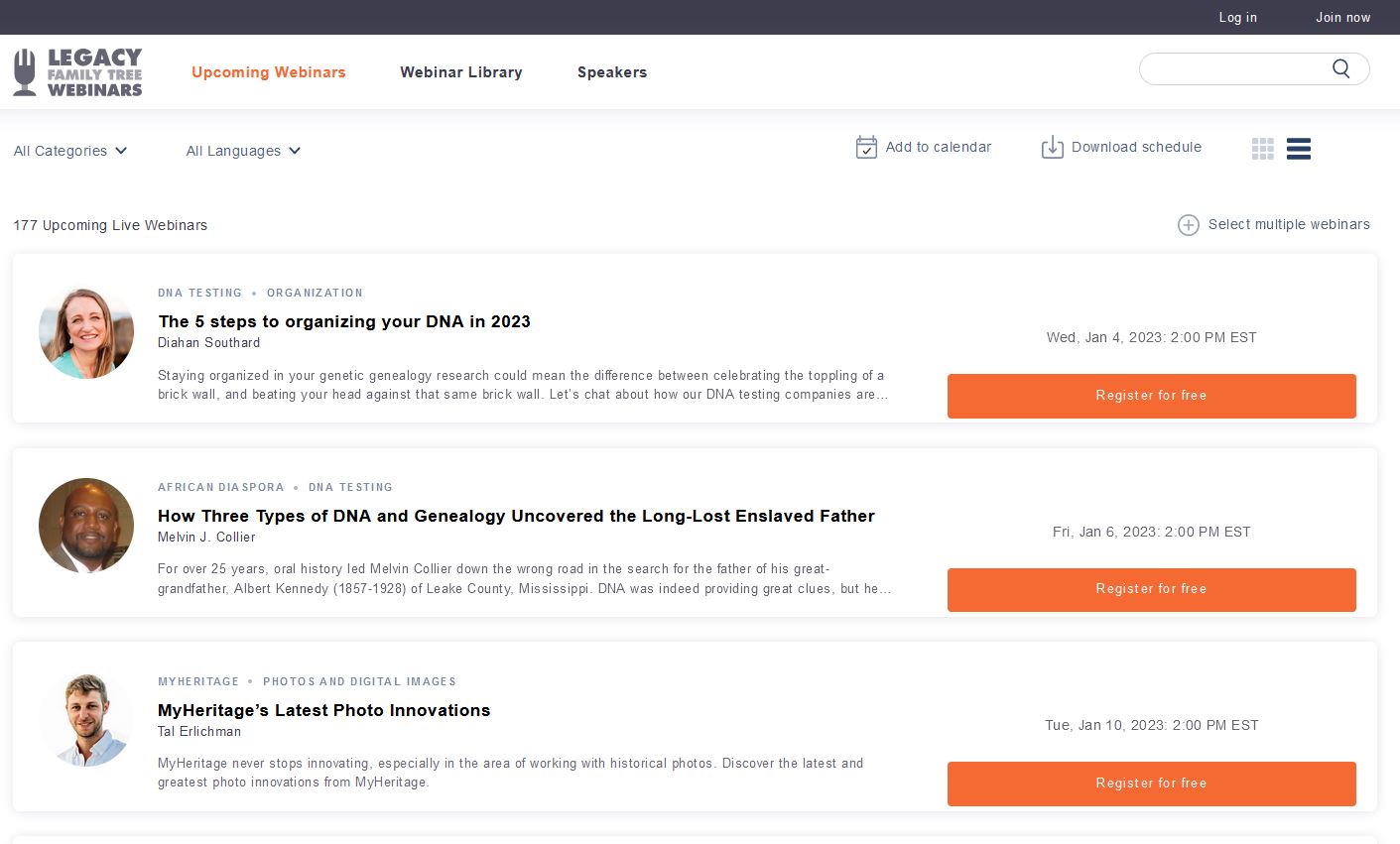This image is a detailed screenshot of the Legacy Family Tree Webinars website. The layout features a mostly white background with prominently displayed black text. A sleek black menu bar spans the top of the page, with options presented in white text. On the upper right corner of this bar, the options to "Login" and "Join Now" are clearly visible.

Situated beneath this are key elements: on the left side, a distinctive microphone logo is adjacent to the bold, capitalized text "LEGACY FAMILY TREE WEBINARS." Just below, a bright orange section highlights "UPCOMING WEBINARS," followed by key options in black text, including "Webinar Library" and "Speakers." Further to the right, there is a functional search bar.

Directly underneath this top section, horizontally arranged from left to right, are dropdown menus labeled "All Categories" and "All Languages," accompanied by convenient action buttons for adding to the calendar and downloading the schedule.

The main content area begins with a header stating "177 Upcoming Live Webinars," alongside a functional button allowing users to select multiple webinars. Below this header, three webinar listings are shown, each featuring a speaker's photo and detailed titles. The webinars are titled as follows, from top to bottom:
1. "The Five Steps to Organizing Your DNA in 2023"
2. "How Three Types of DNA in Genealogy Uncovered the Long-Lost Enslaved Father"
3. "MyHeritage's Last Photo Innovations."